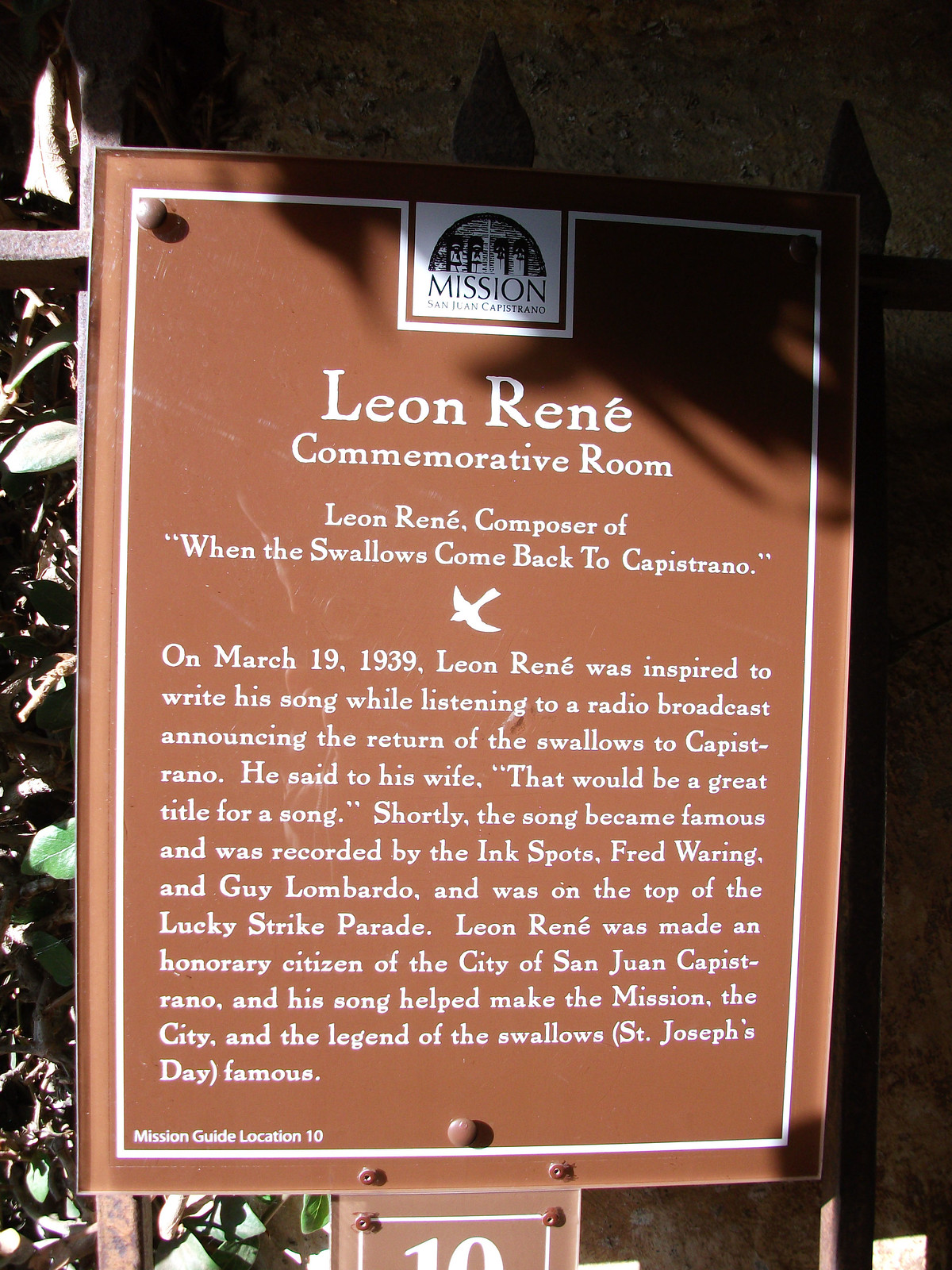The image depicts a brown plaque with a white border, featuring intricate white lettering. At the top, there's a symbol associated with a mission. The sign reads "Leon René Commemorative Room" and continues, "Leon René, composer of ‘When the Swallows Come Back to Capistrano.’" Below this is a small illustration of a white bird. The text further elaborates: "On March 19, 1939, Leon René was inspired to write his song while listening to a radio broadcast announcing the return of the swallows to Capistrano. He said to his wife, 'That would be a great title for a song.' The song soon gained fame and was recorded by the Ink Spots, Fred Waring, and Guy Lombardo, eventually topping the Lucky Strike Parade." The sign also notes that Leon René was made an honorary citizen of San Juan Capistrano and credits his song with boosting the fame of the mission, the city, and the legend of the swallows, celebrated on St. Joseph's Day. At the bottom, it reads "mission guide location number 10," and the sign is set against a backdrop of shrubbery.